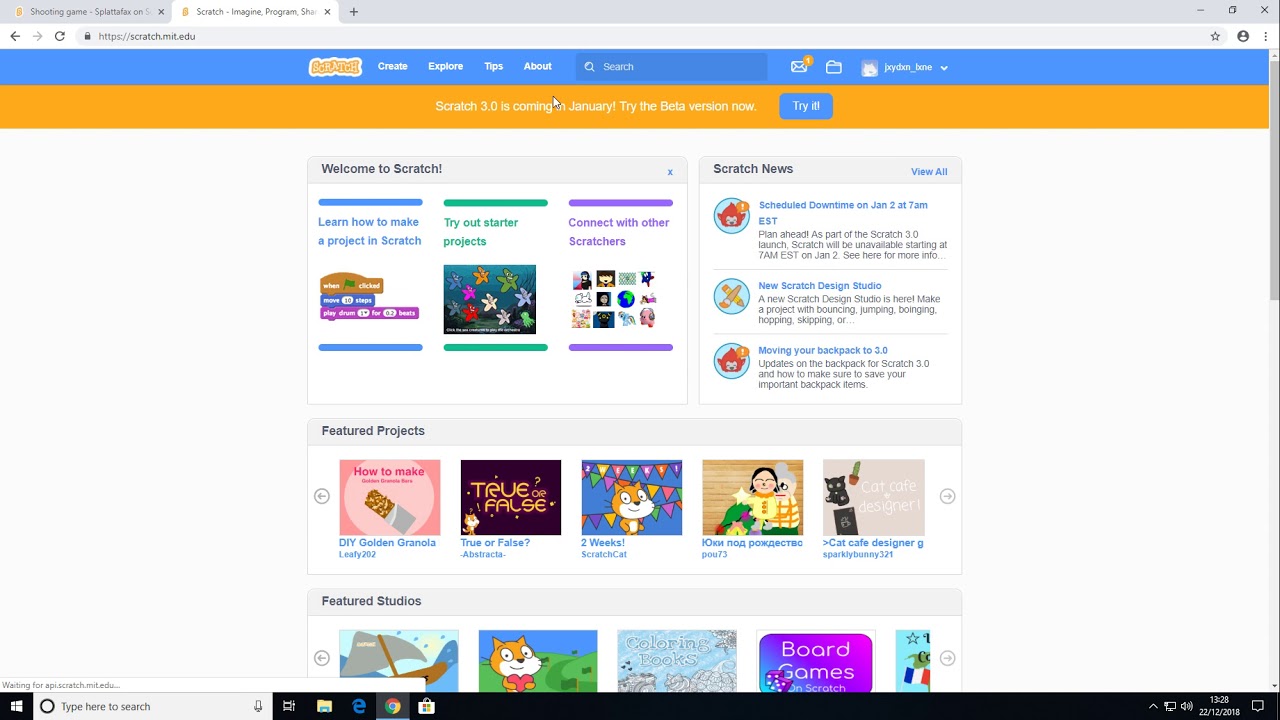This image showcases an open laptop displaying the Scratch website, specifically the URL "scratch.mit.edu." The visible tab on the web browser shows that it's open to the Scratch homepage, where a prominent banner announces "Scratch 3.0 is coming in January. Try the beta version now," accompanied by a blue button labeled "Try it."

In the top-left corner, the page title reads "Scratch - Imagine, Program, Share." Moving further down, a blue navigation bar is visible, containing menu options: "Scratch," "Create," "Explore," "Tips," and "About." To the right of this menu, there's a search icon, a message icon with a notification (indicated by the number '1'), and a folder icon likely for saving projects. Beside these icons, the user profile is shown, labeled "JRYDXN_BNE."

Beneath the navigation bar, the main content of the Scratch page is divided into several sections. The first section welcomes users to Scratch and includes options such as "Learn how to make a project in Scratch," "Try out starter projects," and "Connect with other Scratchers." To the right of this, the page highlights "Scratch News" along with other updates.

Further down, there are sections marked "Scratch Featured Projects" and "Featured Studios," each containing linked boxes that provide additional information and visuals related to their respective topics.

Background elements include another web page open to a shooting game called Splatifax, partly visible behind the current web browser window.